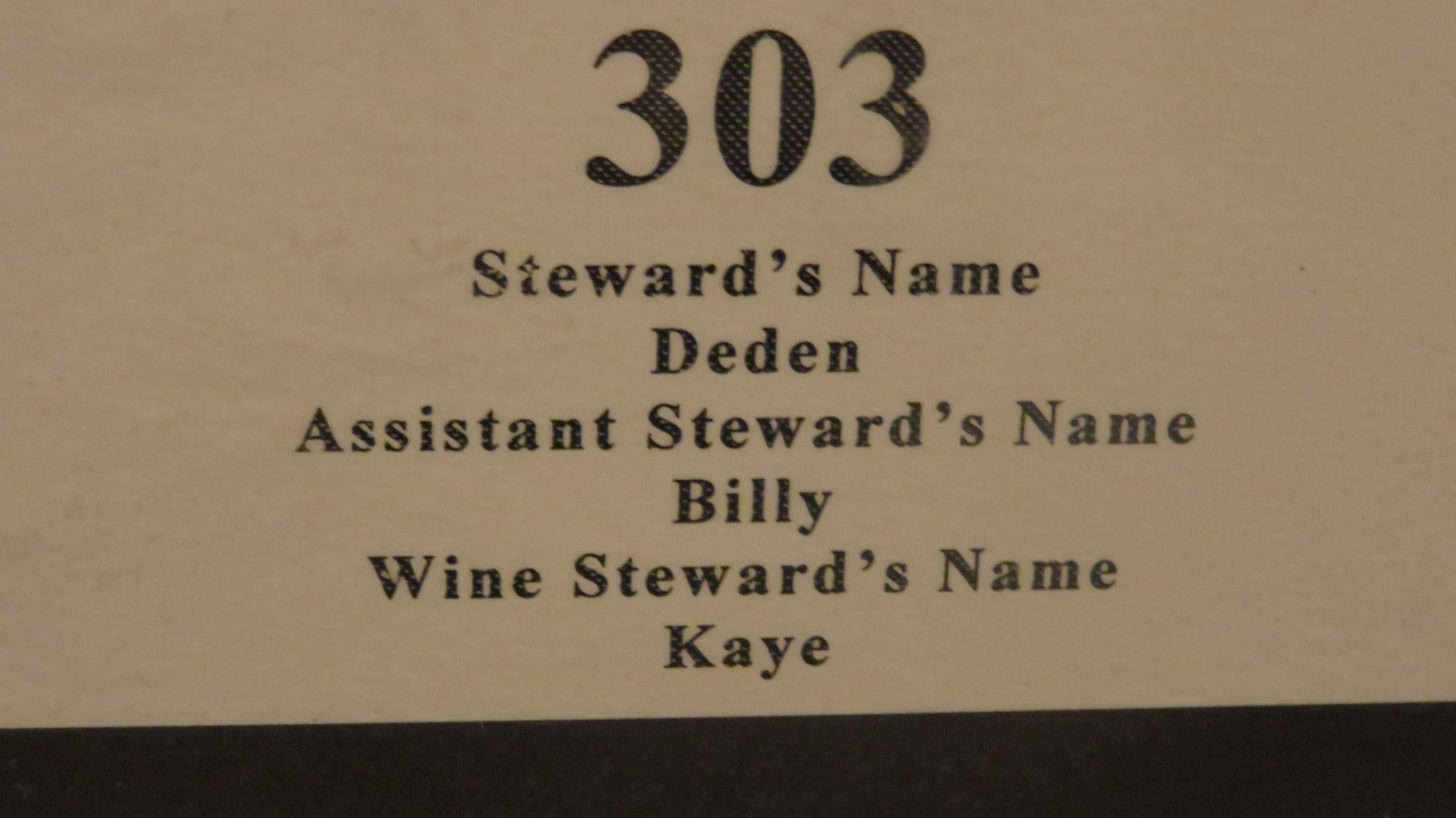The image features a textured, beige background with black text covered in small white polka dots. Dominating the top of the image is the large number "303." Below this, there are three lines of text in a smaller font, listing names and titles: "Steward's Name: Deedan," "Assistant Steward's Name: Billy," and "Wine Steward's Name: Kay." At the bottom of the image, there is a dark gray border stretching from left to right. The overall impression is of a sign or decal displaying these names, possibly indicating a room or a position roster.